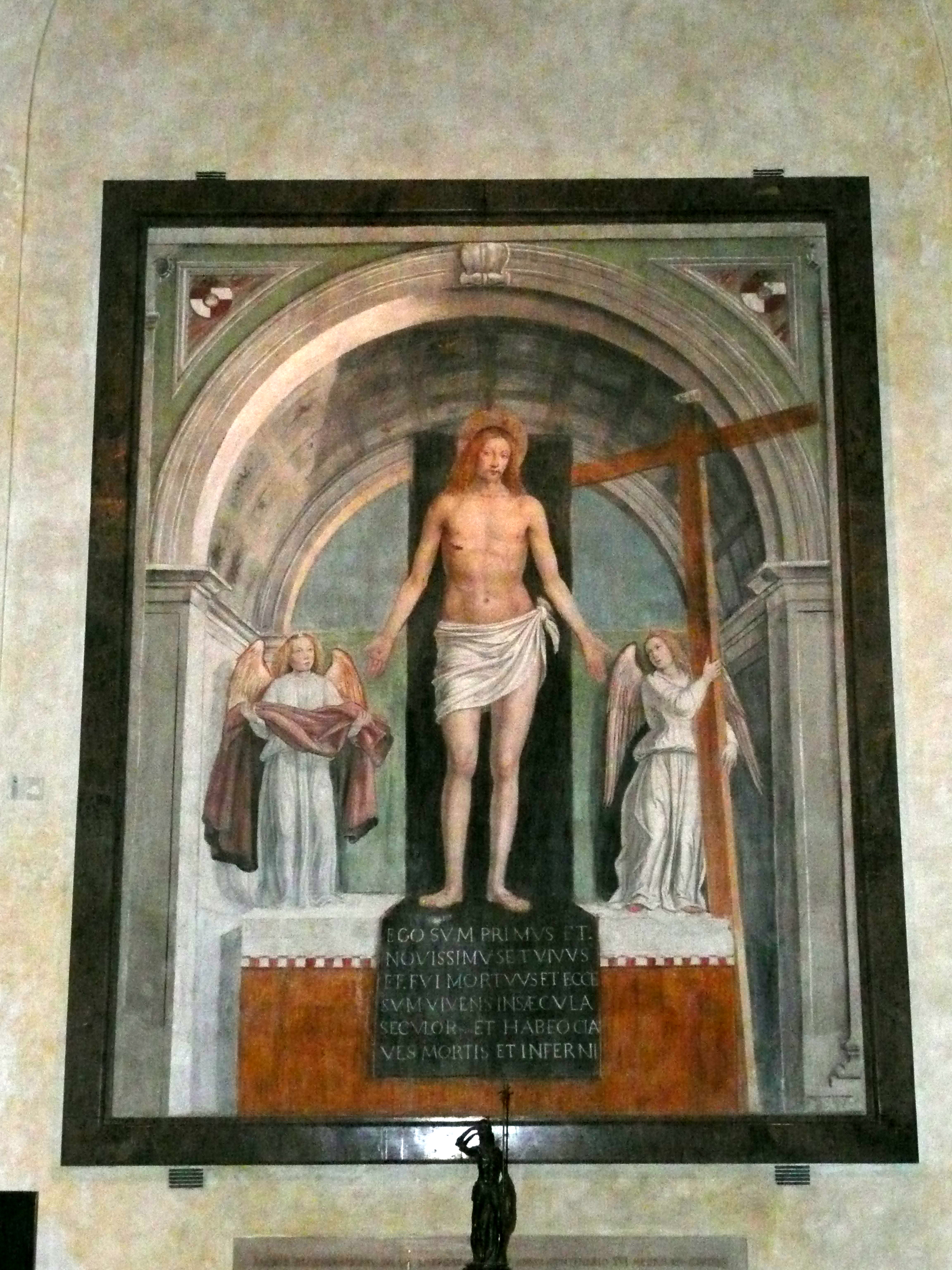This photograph displays a deeply religious painting likely set in a museum or a church, encased in a dark brownish-black frame, and mounted on a cream-colored stone wall with brown patches. The painting, centered under a gray marble archway with a grid-like pattern, depicts a standing figure of Jesus Christ, clad only in a white loincloth or sarong. He is flanked by two angels with closed wings, positioned to the left and right behind him, only reaching up to his waist. The left angel holds a cloth, while the right angel bears a large brown wooden cross. Below Jesus, inscribed in Latin, there is some text, although it is not readable. Additionally, a small black statue is placed beneath this painting on the wall.